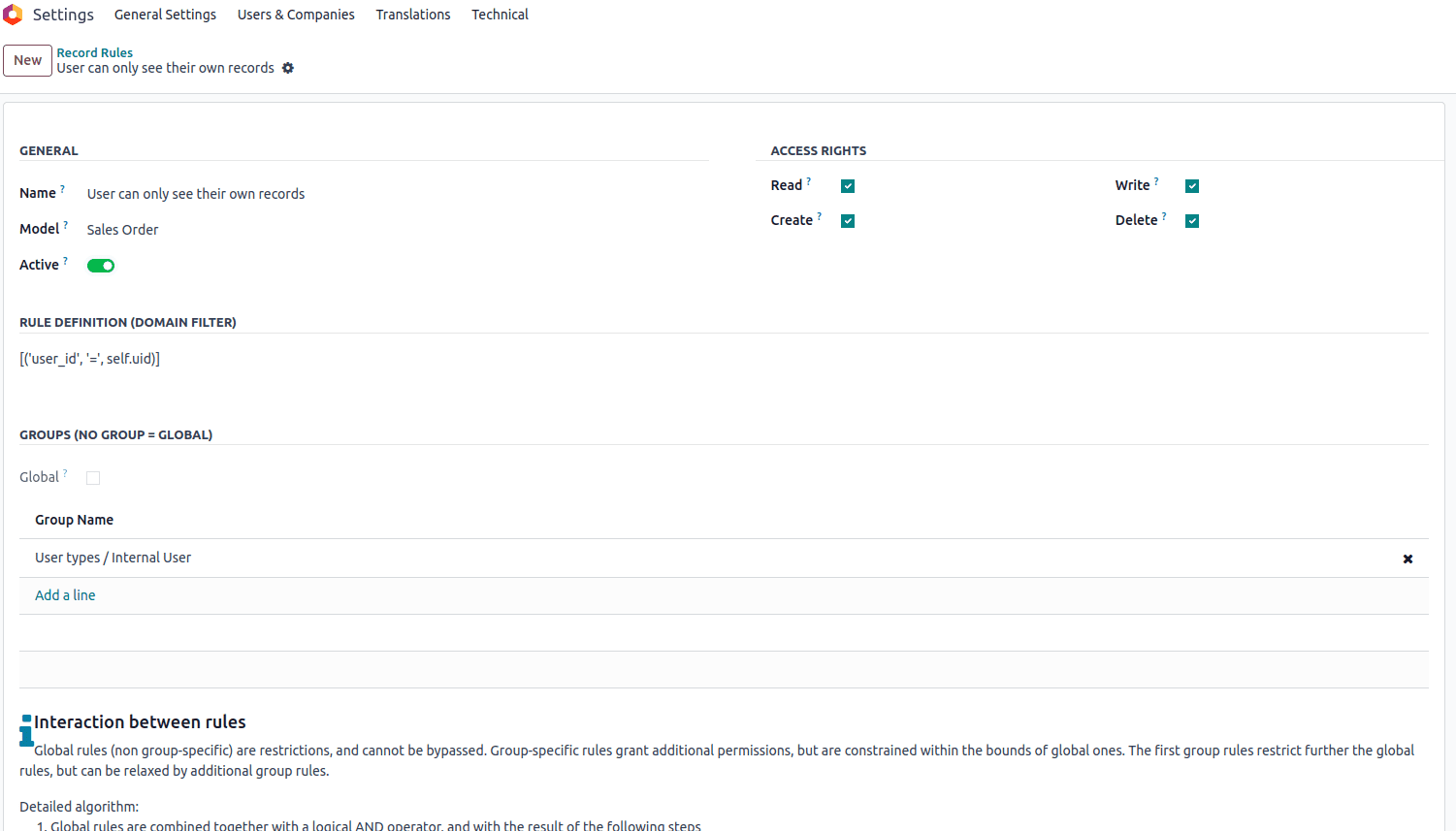This image is a detailed screenshot of a settings page from either a website or a software platform. In the top-left corner, the page is clearly labeled "Settings," and is accompanied by a distinct hexagonal logo composed of three shades of orange and red.

The navigation menu stretches across the top with the following tabs in order: Settings, General Settings, User and Companies, Translations, and Technical. Below this primary menu, there's a prominent button labeled "New." To the right of this button, there's another titled "Record Rules." Additionally, there's a note that reads "User can only see their own records," accompanied by a gear icon symbolizing further configuration options.

"Record Rules" is highlighted in blue, while "New" is presented as a clickable white button.

The page is divided into two main columns: "General" and "Access Rights." Under "General," there are input fields labeled "Name," "Model," and an "Active" status which features a green toggle switch indicating it's enabled. Below these fields is the section "Rule Definition," which includes a "Domain Filter" (written as "Domain Filter" in parentheses for clarity) followed by a concise code snippet or short script relevant to the filter settings.

Overall, this settings page screenshot presents various options for configurations and permissions, with clear labels and interactive buttons for user engagement.